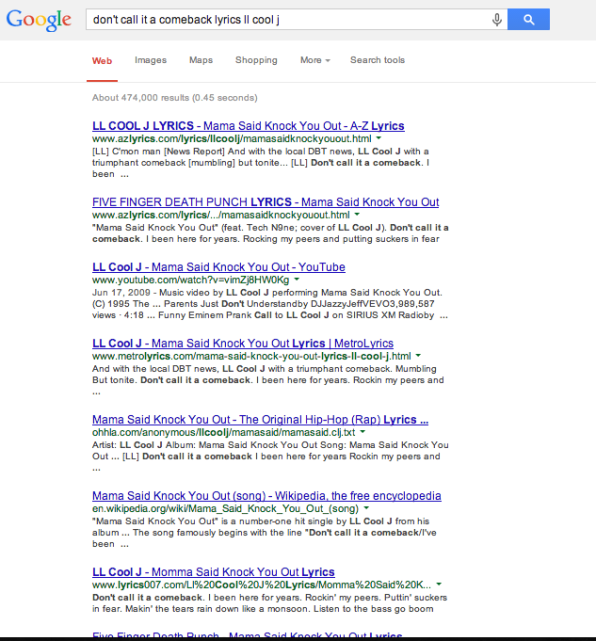The image depicts a screenshot of a Google search results page. The familiar Google logo with its multicolored letters is prominently displayed at the top. In the search box just below the logo, the user has typed "don't call it a comeback lyrics to cool J". 

Beneath the search box, the "Web" category is highlighted in red, signifying that the web search results are being displayed. Other search categories such as Images, Maps, Shopping, More, and Search Tools are also visible but not selected. The screen indicates that there are approximately 474,000 results for the query, retrieved in 0.45 seconds.

The results are structured into eight listings, with the eighth listing partially cut off at the bottom of the screenshot by a black line signifying the page's end. Each result is formatted with a blue clickable link followed by a green URL. For instance, one of the listed links features the title "Mama Said Knock You Out - 'Don't call it a comeback,'" hinting at the relevant lyrics beneath it.